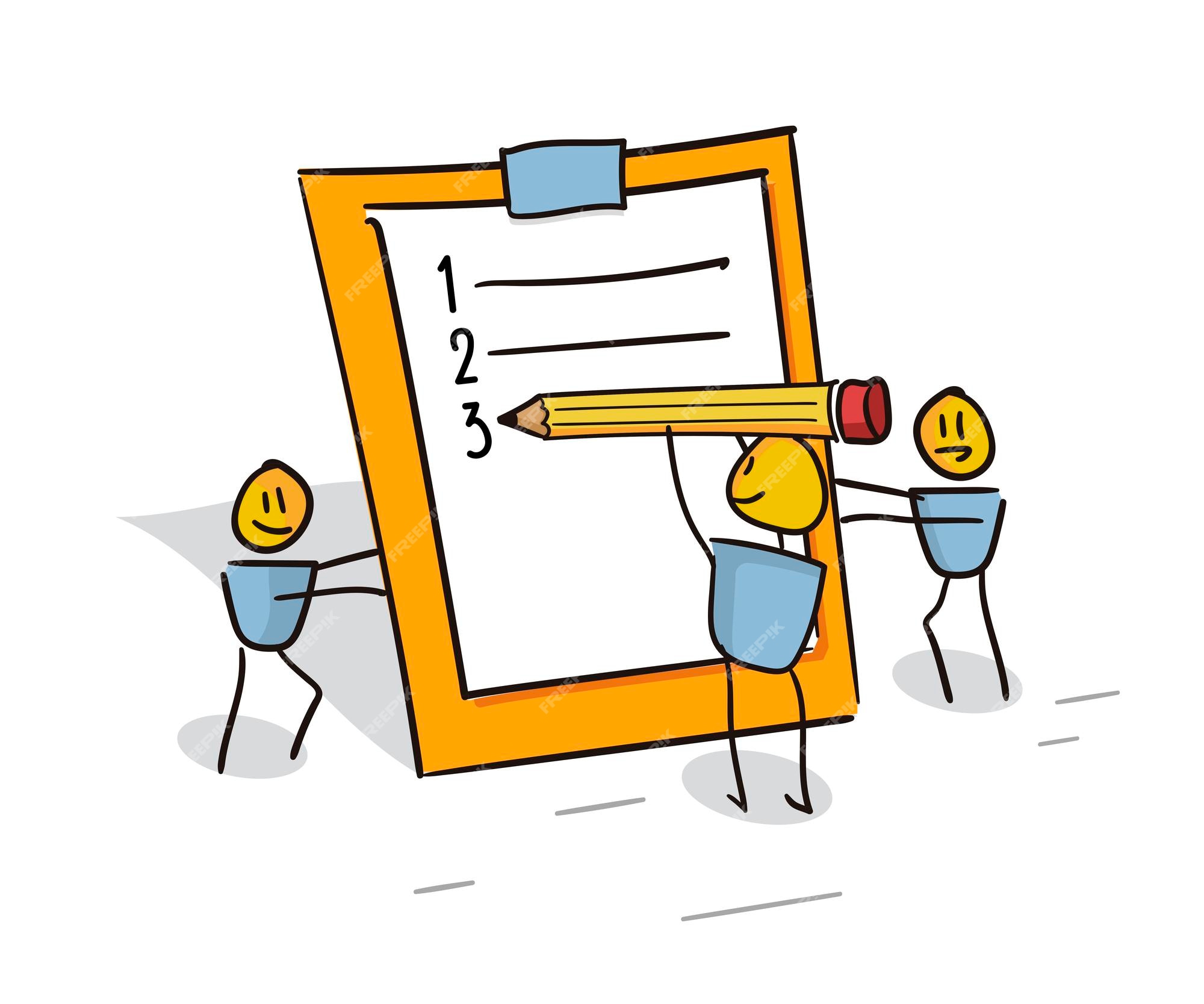This image is a simplistic clipart depiction of a piece of paper with a yellow border and a piece of blue tape at the top center, creating the appearance that it is taped to a wall or board. The inner section of the paper is white and contains three numbered lines: "1," "2," and "3." Accompanying the numbers, three stick figures with yellow faces and blue teacup-shaped bodies are visible. Each stick figure has black lines for eyes and a curved line for a smile, showing their happy expressions. Two of these figures are positioned on either side of the paper, holding it up, while the third figure, standing at the bottom center, grips a large pencil that is about as tall as he is, appearing to write on the paper. A notable detail is the shadow reflection beneath the paper and the stick figures, adding depth to the otherwise flat graphic. The overall scene conveys a collaborative effort among the stick figures as they assist the third figure with his writing task.